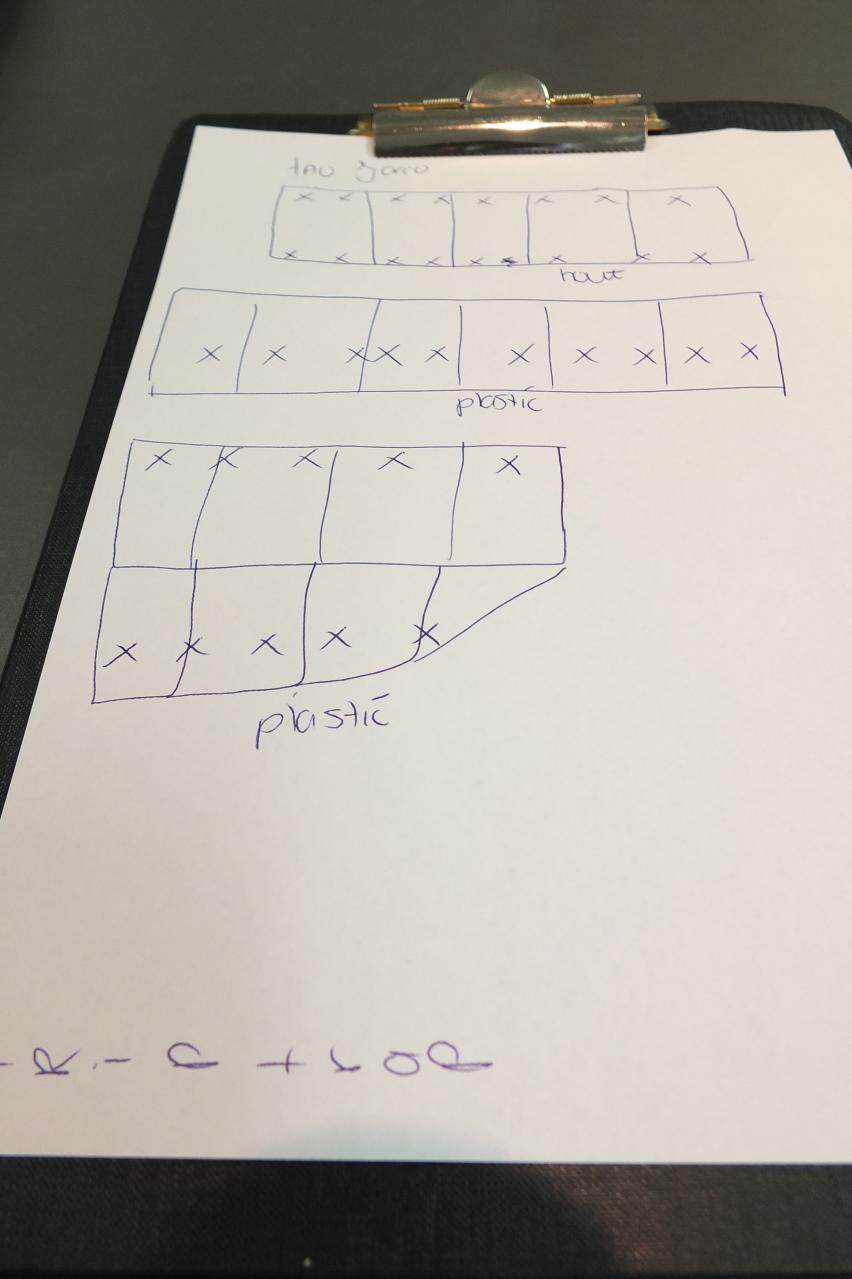This image depicts a detailed hand-drawn diagram or blueprint, presumably for a project in the planning stages. At the bottom of the page, the text "Trip Trap" serves as an indicative title. The diagram itself is organized into three distinct rows, each horizontally aligned with multiple compartments.

The top row features five contiguous square sections, each marked with four X's. Below this, the middle row comprises six joined sections, with two X's in each square. The notation "plastic" is inscribed beneath this row, implying that the material specified for these components is plastic. The bottom row presents the most complex structure: it consists of eight sections, where four are square and one is triangular, all similarly marked with X's. This row also bears the "plastic" label, reinforcing the use of plastic for these sections.

The sketch is rendered on white paper, likely with pen or pencil, and provides a meticulous layout of what appears to be the structural design of the project labeled "Trip Trap."